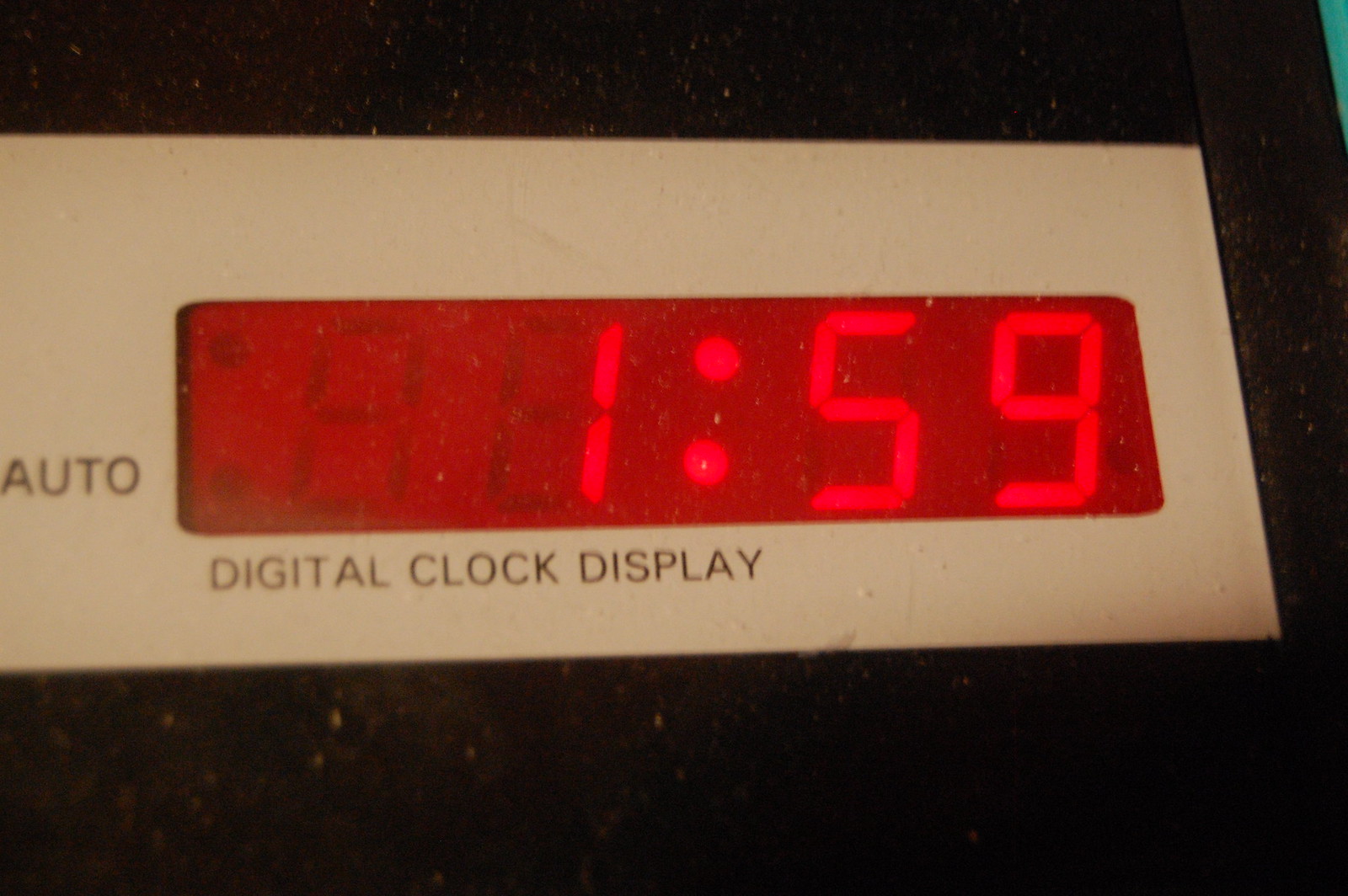This image features a vintage digital clock, likely from the 1970s or 1980s. The clock is predominantly black and has a square frame. The time display is lit in a striking red and currently shows 1:59. To the left of the display, the word "Auto" is visible, while the bottom part of the clock reads "Digital Clock Display." The clock appears to be covered in a fine layer of yellowish dust or pollen, giving it an overall dirty look. The particles are spread across the entire clock, suggesting it may need a thorough cleaning.